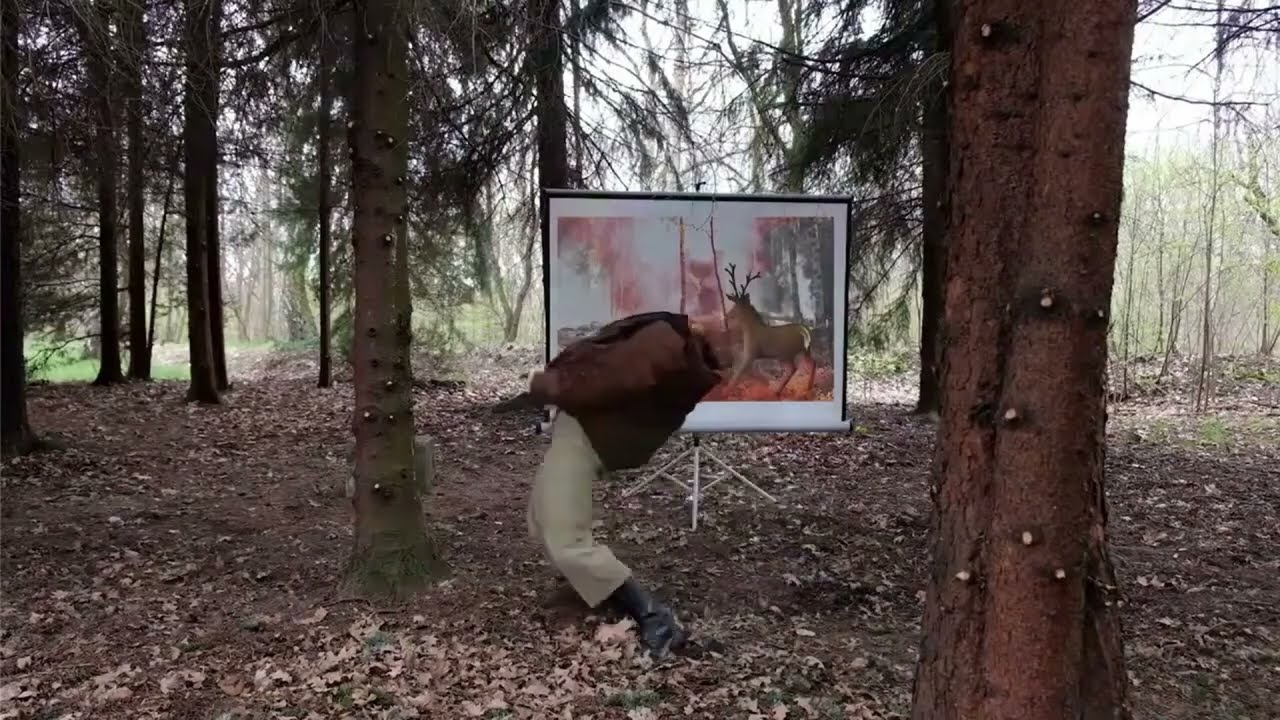This photograph, set in a forested area with brown-trunked pine trees and scattered dead leaves on the ground, presents a surreal scene. A man, dressed in a brown jacket, tan pants, and black footwear, is bending backwards in an exaggerated arch reminiscent of the Matrix's bullet-dodging pose. This action is performed in front of a screen or possibly a painted backdrop, depicting a deer in a forest. Curiously, the man's head appears to be missing, blending seamlessly into the image of the deer behind him, with the head seemingly edited out or disappearing into the deer projection. The surroundings suggest it could be autumn, with a sparse ground cover of primarily dirt and few undergrowth. This intriguing visual suggests a blend of artistic photography and digital editing, creating a mysterious and slightly eerie atmosphere.